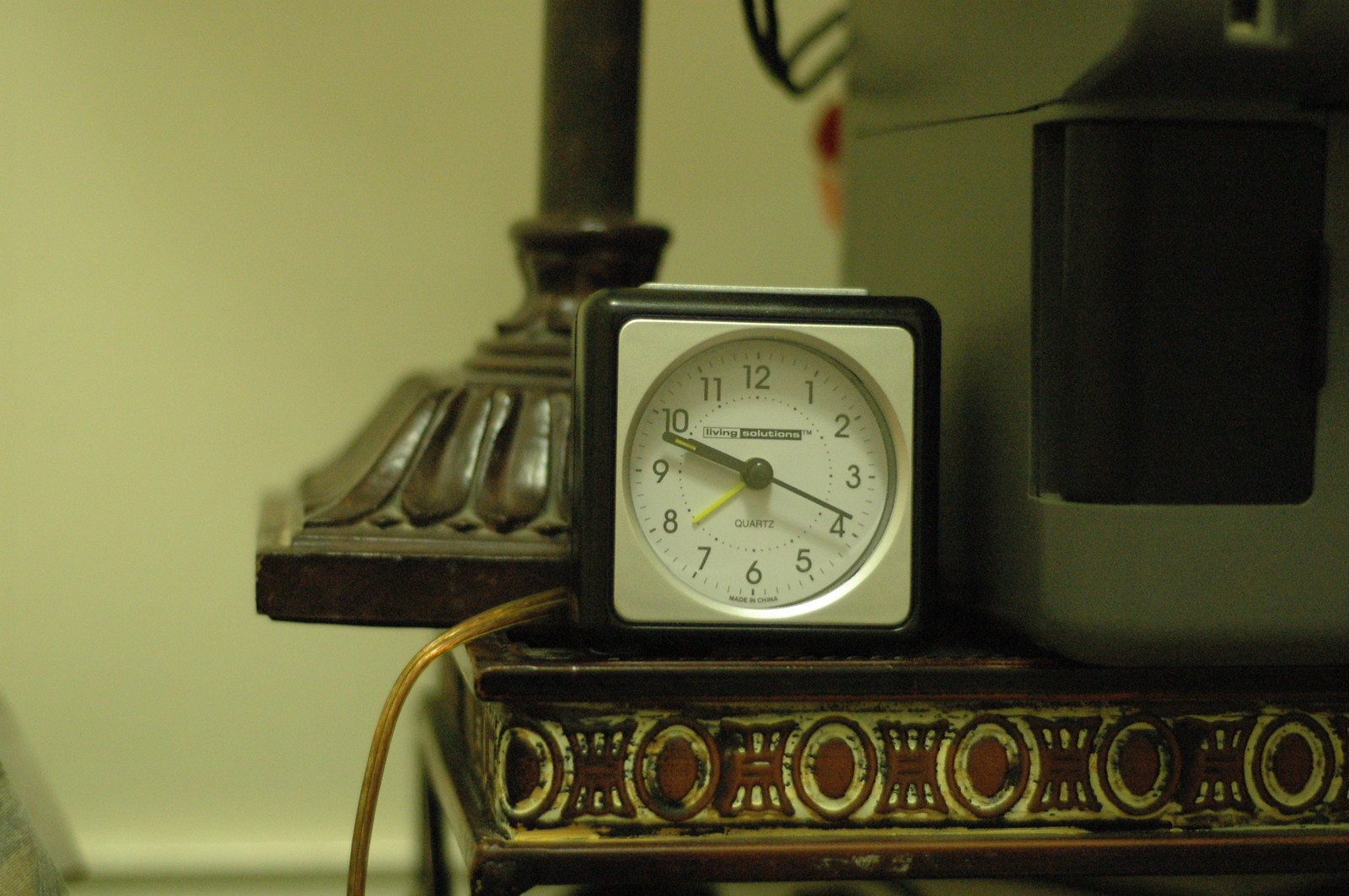The image features a square analog clock with a white face encased in a dark cherry wood frame, resting on a wooden table of similar hue. The round clock face displays all twelve numbers, and it is currently showing the time as 10:19. The clock has three hands: a black hour hand, a black minute hand, and a distinctive yellow second hand, potentially for alarm settings. The table surface exhibits intricate white carvings etched into the dark wood. Behind the clock, partially visible, is the base of a lamp made of solid wood. To the right of the clock, there is a large silver-colored appliance with a black window, which looks like it could be a printer or a similar machine. An orange or greenish copper wire extends from the clock, lying across the table. The combined elements provide a rustic yet functional aesthetic to the scene.